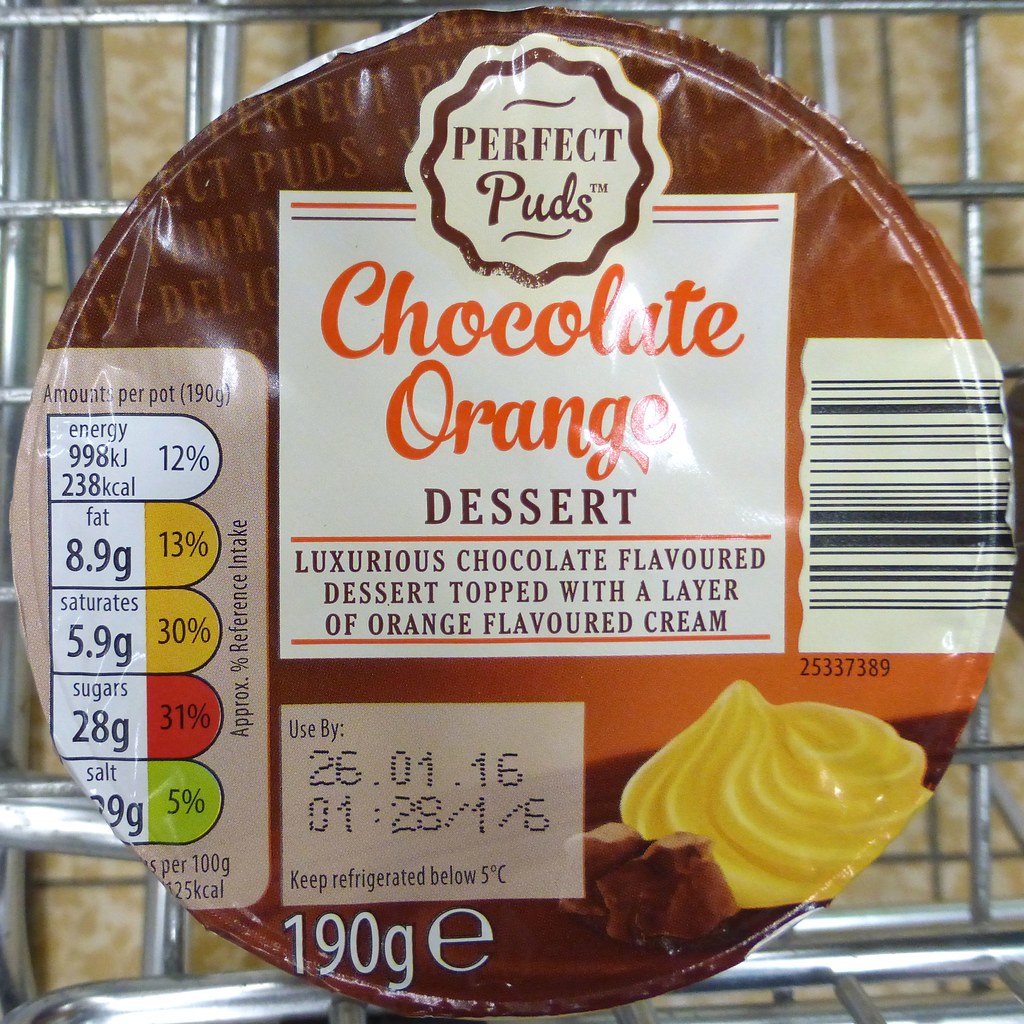The photograph captures a round can of dessert viewed directly from above, set against the aluminum or steel rods of a shopping cart. The can features the "Perfect Puds" trademark prominently on the top cover. The label reads "Perfect Puds Chocolate Orange Dessert," described as a "Luxurious chocolate-flavored dessert topped with a layer of orange-flavored cream." The packaging includes a visual of the dessert, depicting a chocolate slice with a swirl of orange cream, adding to its appetizing appeal. Additional details on the can include a use-by date of "26.01.16" and storage instructions to keep it refrigerated below 5 degrees Celsius. Nutritional information, such as "8.9 grams of fat," is listed on the side.